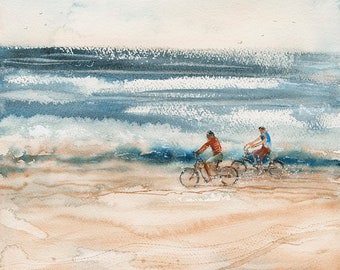This captivating watercolor painting depicts a serene beach scene featuring two figures bicycling along the shoreline. The canvas, relatively small in size, showcases a vibrant contrast between the tranquil yellow-orange sands and the dynamic blue hues of the ocean waves. The sky above is predominantly white, perhaps signifying a bright or overcast day.

In the foreground, the two cyclists, who appear to be men, are positioned just beside the edge of the beach where the waves crash. One rider, situated slightly right of center, dons a red shirt with gray pants and rides a reddish-black bicycle. He has black hair and no helmet. The other cyclist, wearing a white cap, is clothed in a bluish shirt and red pants, pedaling a mostly black bicycle. Both figures are framed against the backdrop of powerful waves, depicted in a mix of whites and dark blues, creating a vivid sense of movement as they roll towards the shore.

Tracks in the sand trail behind the bicycles, adding to the realism and narrative of the scene. The beach stretches from one side of the painting to the other, capturing the expanse of the shoreline and the moment's tranquility amid the relentless energy of the ocean.